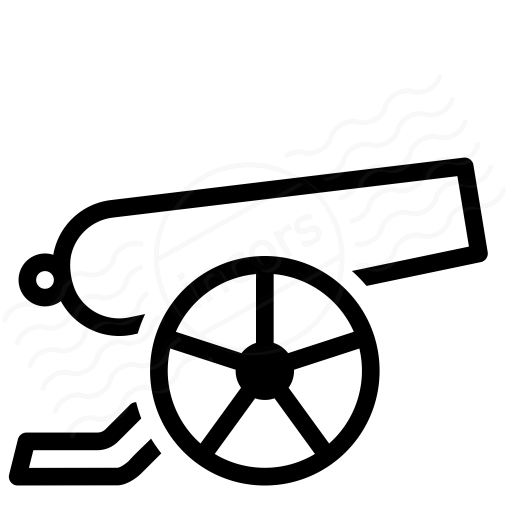The image depicts a minimalist, black-ink line drawing of an old-fashioned cartoon cannon on a white background. The cannon is composed of several distinct parts, including a slightly upward-tilted barrel pointing towards the right, a ball likely representing a cannonball, and an ignition chamber, each delineated with bold black lines. The cannon is mounted on a wheel situated towards its left, featuring an inner center disc with five spokes leading to the rim. Notably, the body of the cannon does not intersect with the wheel. A resting base supports the wheel to prevent it from rolling away. A faint gray watermark, consisting of a circle with wavy lines and partially obscured text, overlays the image.